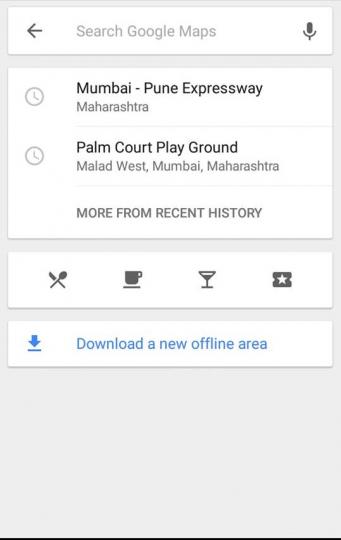In the screenshot of a phone interface, the top section features a search bar with gray text that reads "Search Google Maps." On the left, there is a left arrow, and on the right side of the search bar, there is a microphone icon. Below the search bar, a white rectangular area displays location information, including "Mumbai Poon Expressway, Maharashtra" and "Palm Court Playground, Malad West, Mumbai, Maharashtra," followed by the phrase "more from recent history."

Beneath this section, another white rectangle contains a series of four icons, each set within a circle. From left to right, the icons depict a crossed knife and spoon, a coffee cup, a goblet, and a ticket with a star in the center.

Further down, there is another section that includes a link reading "Download a New Offline Area" accompanied by a download symbol on the right side. The entire interface is set against a light gray background, providing a clean and organized layout.